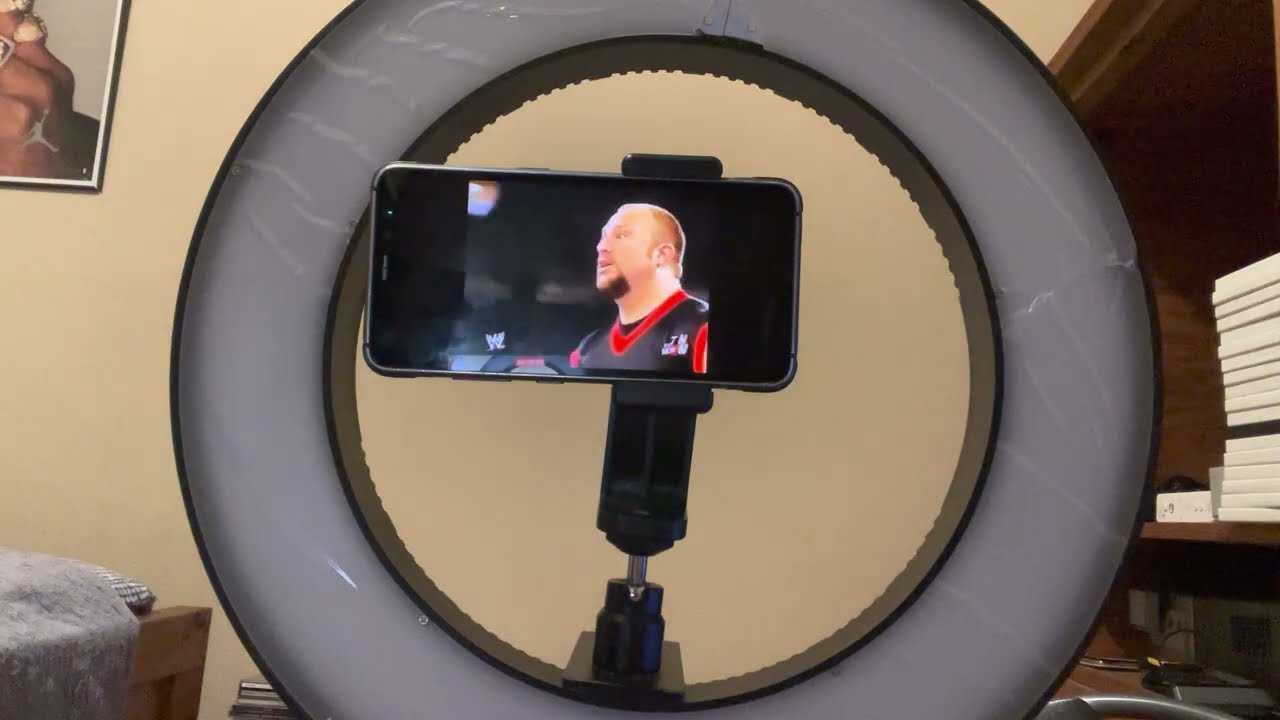The photograph depicts a detailed interior scene, ostensibly an office space with a tan or beige wall in the background. Central to the image is a circular lamp, possibly used for lighting during phone-based video calls, indicated by the stand with a mounted cell phone on its rim. The phone displays an image of Bubba Ray Dudley from the WW network, appearing poised to perform a wrestling move. On the right side of the frame, there is a brown bookcase. The top shelf of the bookcase holds a row of white books, while the second shelf partially showcases a gray structure. 

Towards the lower left, a desk or possibly a bed with a gray blanket draped over its brown edge can be seen. Adorning the upper left corner of the wall is a framed piece of artwork. This artwork features an orange figure and an iconic image of Michael Jordan performing a slam dunk, and is bordered by a white frame. The photograph is rich in details, creating a layered and dynamic depiction of a living or working space filled with personal and professional elements.